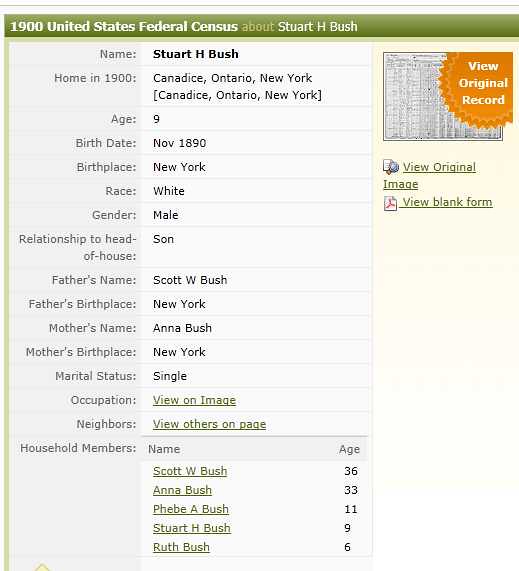The image appears to be a screenshot of a webpage displaying details from the 1900 United States Federal Census about a person named Stuart H. Bush. The webpage has a green border at the top, with a heading that reads, "1900 United States Federal Census about Stuart H. Bush." On the top right corner, there is an orange link labeled, "View original record," along with links at the bottom for "View original image" and "View blank form." 

The main section of the page details the personal and household information of Stuart H. Bush. His home in 1900 is listed as Kandace, Ontario, New York. He was 9 years old, having been born in November 1890 in New York. Stuart H. Bush is described as a white male and a son in the household. His father's name is Scott W. Bush, aged 36, born in New York, and his mother's name is Anna Bush, aged 33, also born in New York. Stuart is noted to be single. 

The household members listed include Scott W. Bush, Anna Bush, Phoebe A. Bush (11 years old), Stuart H. Bush (9 years old), and Ruth Bush (6 years old). There are clickable options for viewing the occupation, neighbors, and other related pages, which suggest additional data linked to this profile.